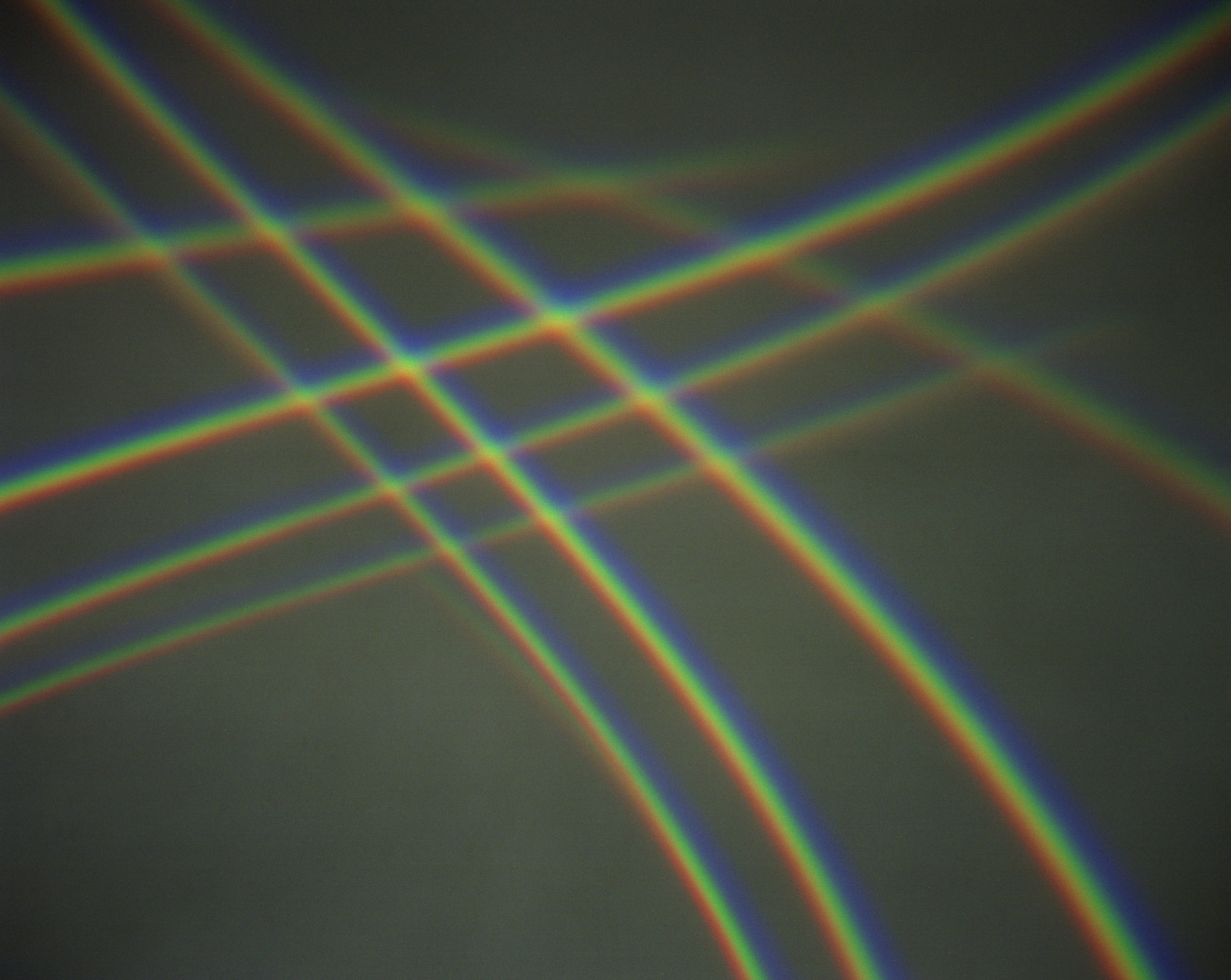The image depicts a series of vividly colored, intertwining lines creating a dynamic and intricate visual effect. There are two primary sets of lines: one set comprises four lines extending from the mid-left edge to the upper right corner, while the other set includes three lines spanning from the bottom right corner to the top left corner. Each line showcases a gradient of rainbow colors, vividly displaying blue, green, yellow, and red hues. These colorful lines intersect in the middle, forming a complex checkerboard or basket weave pattern. The lines appear slightly wavy, contributing to a digital, glitchy aesthetic. The background is a matte gray color, which enhances the vibrancy of the lines and the overall visual impact of the image.